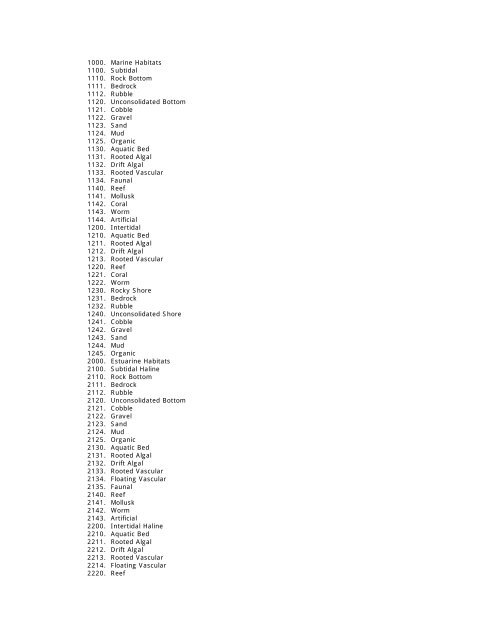The webpage features a simplistic design with a white background and an extensive list of black text entries, each accompanied by numerical codes. Here is the detailed breakdown:

- **Marine Habitats (1000)**: 
  - 1100: Subtitle
  - 1110: Rock Bottom
  - 1111: Bedrock
  - 1112: Rubble
  - 1120: Unsolicited Bottom
  - 1121: Cobble
  - 1122: Gravel
  - 1123: Sand
  - 1124: Mud
  - 1125: Organic
  - 1130: Aquatic Fed
  - 1131: Rooted Algal
  - 1132: Drift Algal
  - 1133: Rooted Vascular
  - 1134: Faunal
  - 1140: Reef
  - 1141: Mollusk
  - 1142: Coral
  - 1143: Worm
  - 1144: Artificial
- **Title Entry (1200)**:
  - 1210: Aquatic Fed
  - 1211: Rooted Algal
  - 1212: Drift Algal
  - 1213: Rooted Vascular
  - 1220: Reef
  - 1221: Coral
  - 1222: Worm
  - 1230: Rocky Shore
  - 1231: Bedrock
  - 1232: Rubble
  - 1240: Unsolicited Shore
  - 1241: Cobble
  - 1242: Gravel
  - 1243: Sand
  - 1244: Mud
  - 1245: Organic
- **Estuarine Habitats (2000)**:
  - 2100: Subtitle Haline
  - 2110: Rock Bottom
  - 2111: Bedrock
  - 2112: Rubble
  - 2120: Unsolicited Bottom
  - 2121: Cobble
  - 2122: Gravel
  - 2123: Sand
  - 2124: Mud
  - 2125: Organic
  - 2130: Aquatic Fed
  - 2131: Rooted Algal
  - 2132: Drift Algal
  - 2133: Rooted Vascular
  - 2134: Floated Vascular
  - 2135: Faunal
  - 2140: Reef
  - 2141: Mollusk
  - 2142: Worm
  - 2143: Artificial
- **Intertidal Haline (2200)**:
  - 2210: Aquatic Red
  - 2211: Rooted Algal
  - 2212: Drift Algal
  - 2213: Rooted Vascular
  - 2214: Floated Vascular
  - 2220: Reef

Each section is categorized with increasing specificity, detailing various marine and estuarine environments as well as intertidal zones, using a structured numerical system to delineate the different habitat types and features.